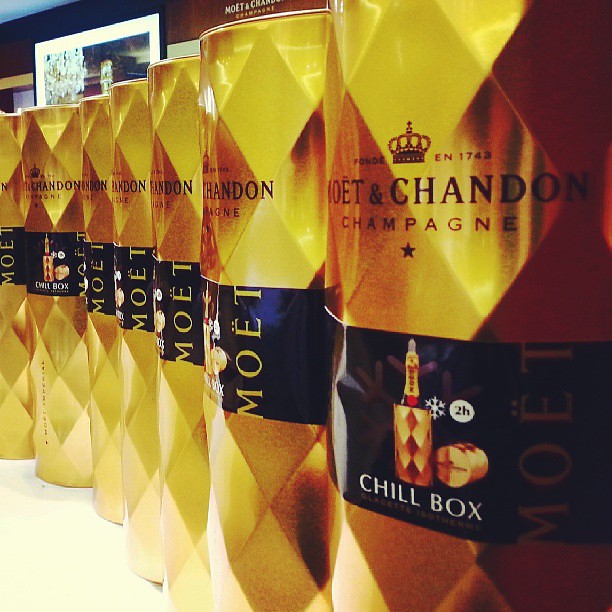This image features a lineup of seven Moet and Chandon champagne bottles stacked side-by-side, all prominently displayed against a minimal backdrop. Each golden-hued bottle is adorned with a black label featuring the iconic crown illustration and inscriptions including "EN 1743" and "Moet and Chandon Champagne Fondé." Additionally, there is a label across each bottle depicting a "chill box," a container designed to keep the champagne cool for two hours, with an accompanying white snowflake symbol. The bottles' wrapping exhibits a geometric diamond design in hues of purplish or dark blue. The photo is taken so closely that the bottles dominate the image, though a picture is visible in the top left corner. The setup implies depth by arranging the bottles in a diagonal line from the bottom right upward, suggesting a retail or promotional setting, potentially within a Moet and Chandon store or headquarters, indicated by inscriptions on the wall in the background.